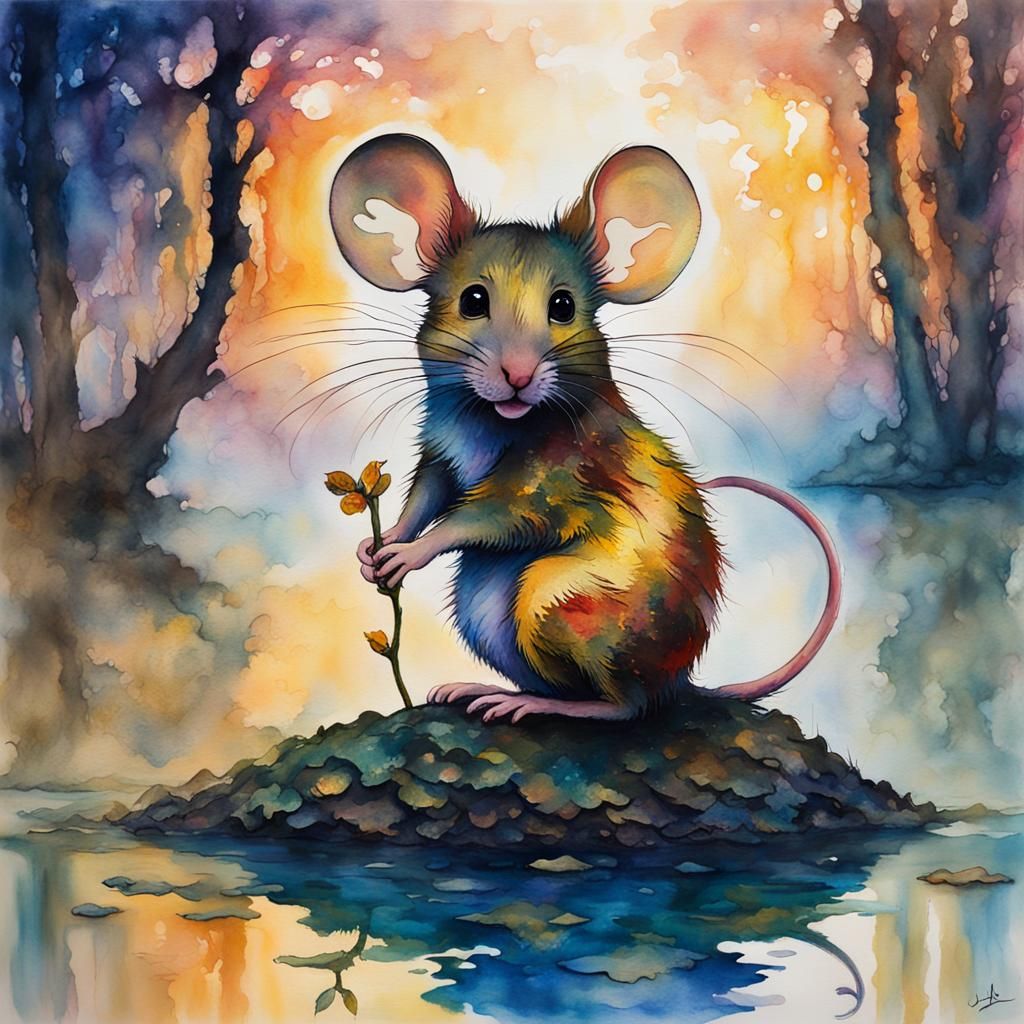This is a detailed digital watercolor painting of a large, whimsical mouse that is front and center in the composition, appearing to stand or sit on its hind legs atop a small pile of rocks or leaves in the middle of a body of water. The mouse, with a colorful coat resembling autumn leaves—brown, yellow, red, and white on its belly—holds a delicate yellow flower or twig with leaves in its small, detailed hands. Its long tail is artistically curled, complementing its large ears which feature intricate white squiggly patterns, adding a whimsical distraction. The mouse's face is endearingly expressive, with numerous whiskers and dark, open eyes. The background portrays a serene, swamp-like landscape with trees on either side and an overall gradient of purples, oranges, and reds, perhaps suggesting a sunset or autumn setting. The reflection of the rock pile in the water adds depth to the artwork, enhancing its enchanting and serene atmosphere.